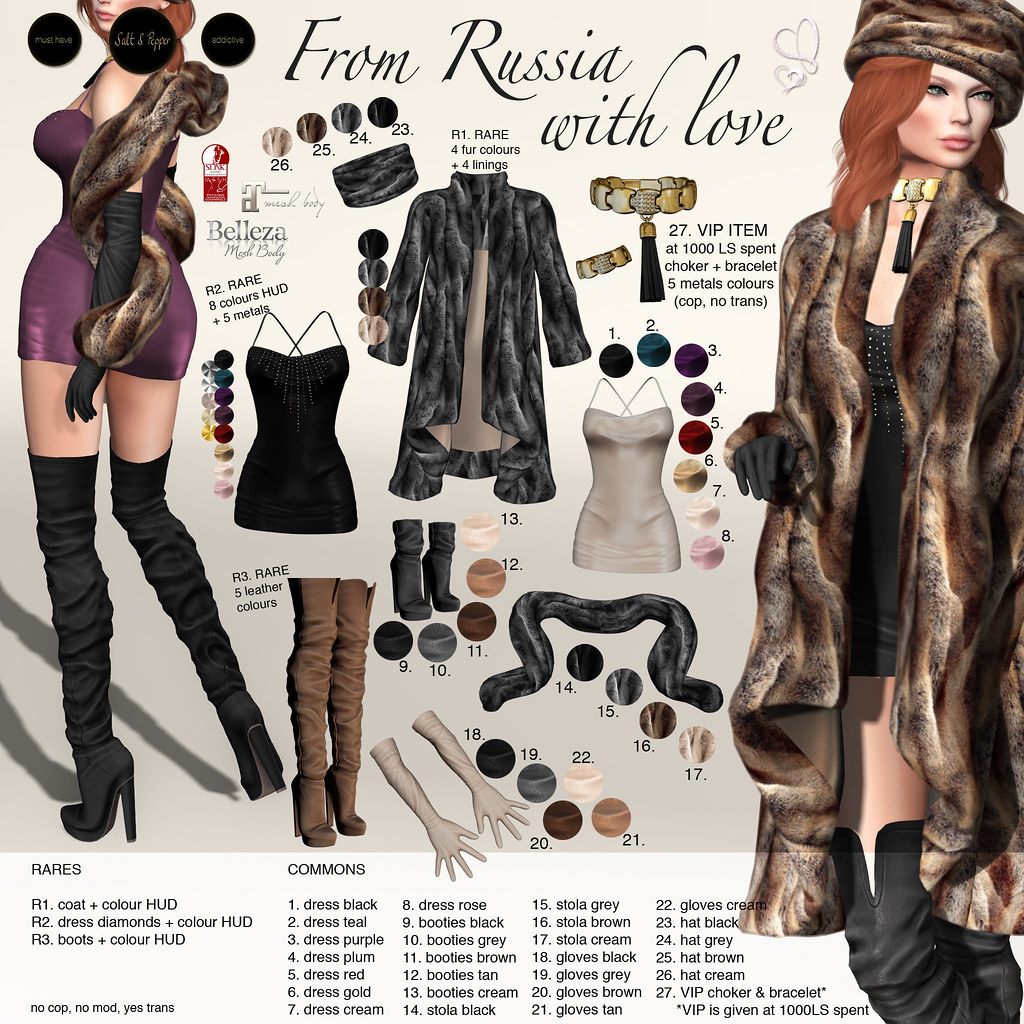The advertisement for a computer game's clothing features a crisp, white background with black, slightly cursive text at the top reading, "From Russia with Love," accompanied by small gray hearts. The ad showcases two AI-generated models. The model on the left is wearing a thigh-high heeled boots ensemble with a short purple dress, a brown stole, and black over-the-elbow gloves. She is posed with her back to us, looking over her left shoulder. The model on the right sports thigh-high black boots, a short black dress, a gold choker with a black tassel, and black gloves paired with a brown fur jacket and red hair. Centered between the two models are various fur and winter clothing items, including a fur scarf, long-sleeve fur coat, mini skirts, and various accessories available in different colors. Below the items, black text organizes the pieces by rarity with 'Rares' labeled R1 coat plus color HUD, R2 dress diamonds plus color HUD, R3 boots plus color HUD, and 'Commons' as dress black (1), dress teal (2), dress purple (3), dress plum (4), dress red (5), dress gold (6), dress cream (7). Additional labels indicate no copy, no modify, and yes transfer capabilities. The layout includes multiple columns detailing all available items and their variations.